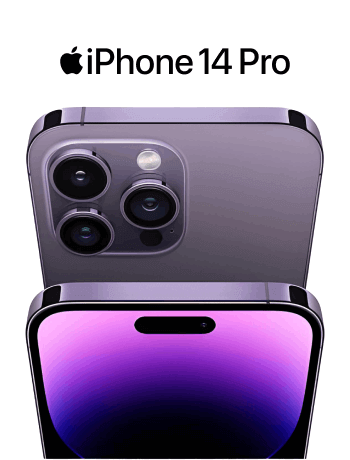A promotional image features the iconic Apple symbol followed by the text "iPhone 14 Pro." Below this, a detailed depiction of the iPhone 14 Pro in a striking purple shade appears. The image showcases both the front and the back of the phone.

The rear view highlights a squared camera module with rounded corners, containing three lenses and a smaller white circle, likely a flash, along with some black spots. The phone's back is a dark purple color, while the top portion appears in a lighter purple hue.

The front view presents a gradient display that transitions from pink at the top to deep blue and black towards the bottom. A prominent black rectangle is situated at the top of the screen, extending to a point on one side. The screen is bordered by a black frame that becomes thicker at the bottom. Additionally, there are two black points and a thin gray line along the top edge of the phone.